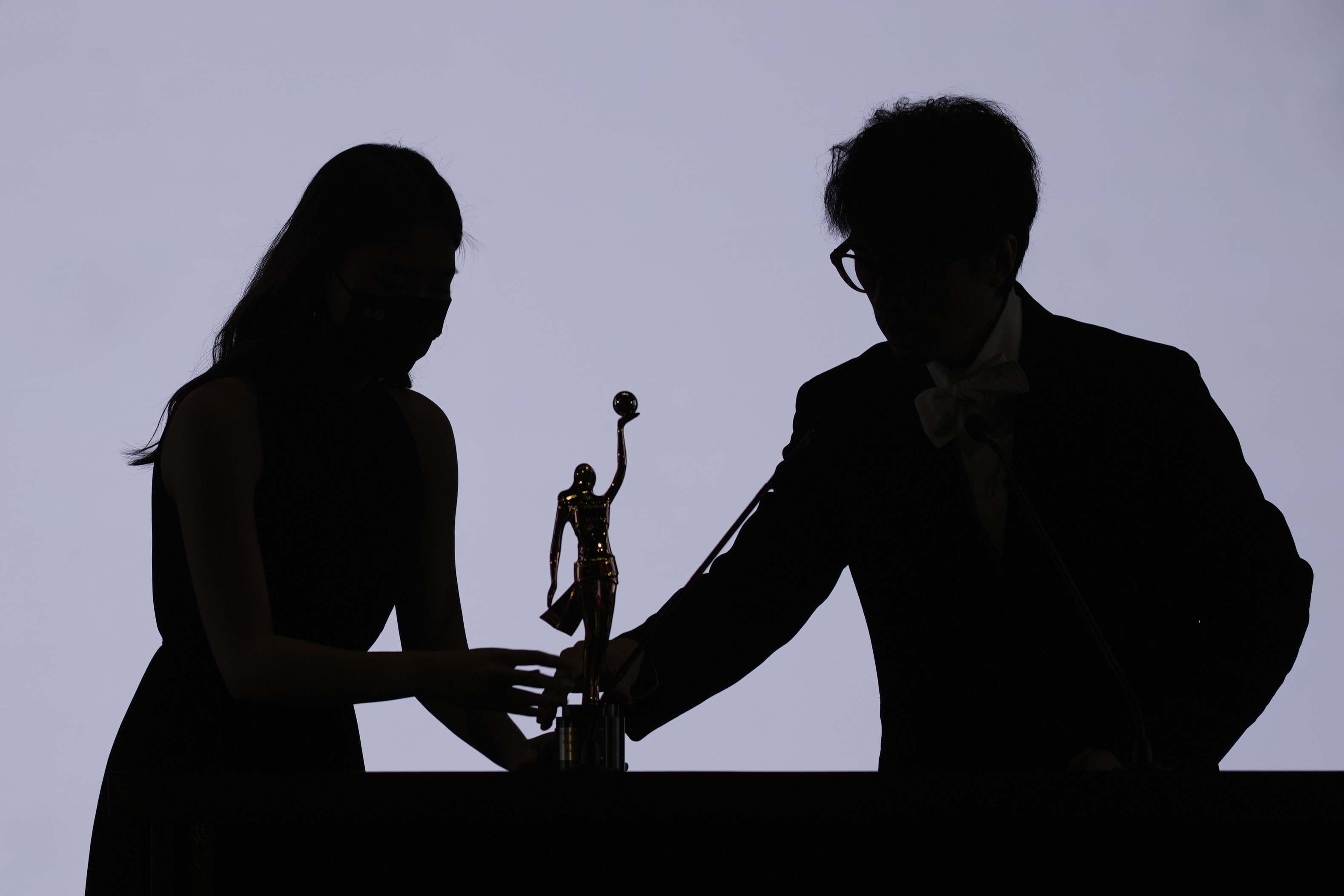This is an artistic, digitally created image featuring the silhouettes of a man and a woman standing closely together against a light purplish-gray background. Both silhouettes appear entirely black, and the man, slightly taller and on the right, is distinguishable by his glasses and a suit-like sharpness in his shoulder outline. The woman, on the left, has long, possibly shoulder-length hair and is likely wearing a dress based on the shadow's shape. They're both reaching out towards a small trophy situated between them. The trophy appears to be a statue of a woman in a dress, her skirt flaring to the left, with one arm raised and holding a ball or similar object. The couple's right hands are extended towards the trophy, creating a scene of connection and shared focus on the central object. The photo is horizontal and rectangular in shape, with no visible text or words adding to its simplicity and elegance.